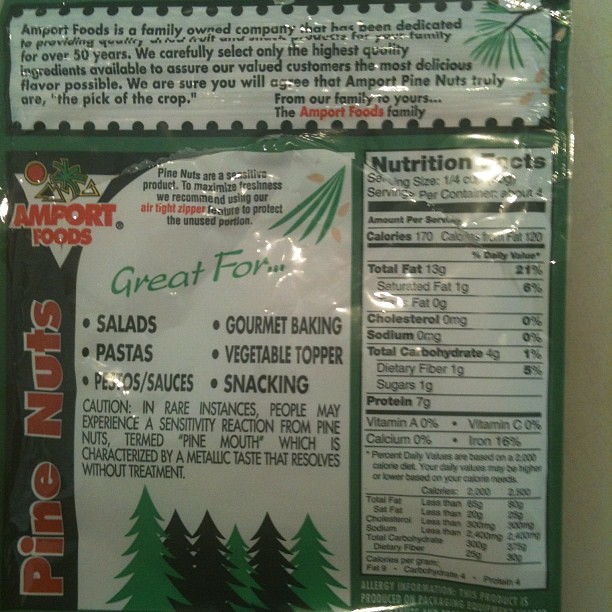This image showcases the back of a package of pine nuts from Amport Foods, a family-owned company dedicated to providing quality products. The package, predominantly green and white with red accents, features various informative sections. At the top, there's a description of the company, emphasizing their commitment to sourcing the highest quality ingredients to ensure exceptional flavor. The name "Amport Foods" is written in black lettering, affirming the family-owned heritage.

The nutritional facts, found on the right side, indicate that a serving size is a quarter cup, with each serving containing 170 calories. The relatively small package holds four servings in total. Central to the package is a list of suggested uses for pine nuts, including salads, pasta, pesto sauces, gourmet baking, vegetable toppings, and snacking.

Additionally, the package includes a cautionary note about "pine mouth," a rare condition that could cause a temporary metallic taste. The visual design of the package features vibrant imagery of pine trees, enhancing its natural pine aesthetic. The words "pine nuts" are prominently displayed on the left side in red lettering against a black background, standing out against the green and white theme. The package also advises zipping the bag closed after use to maintain freshness.